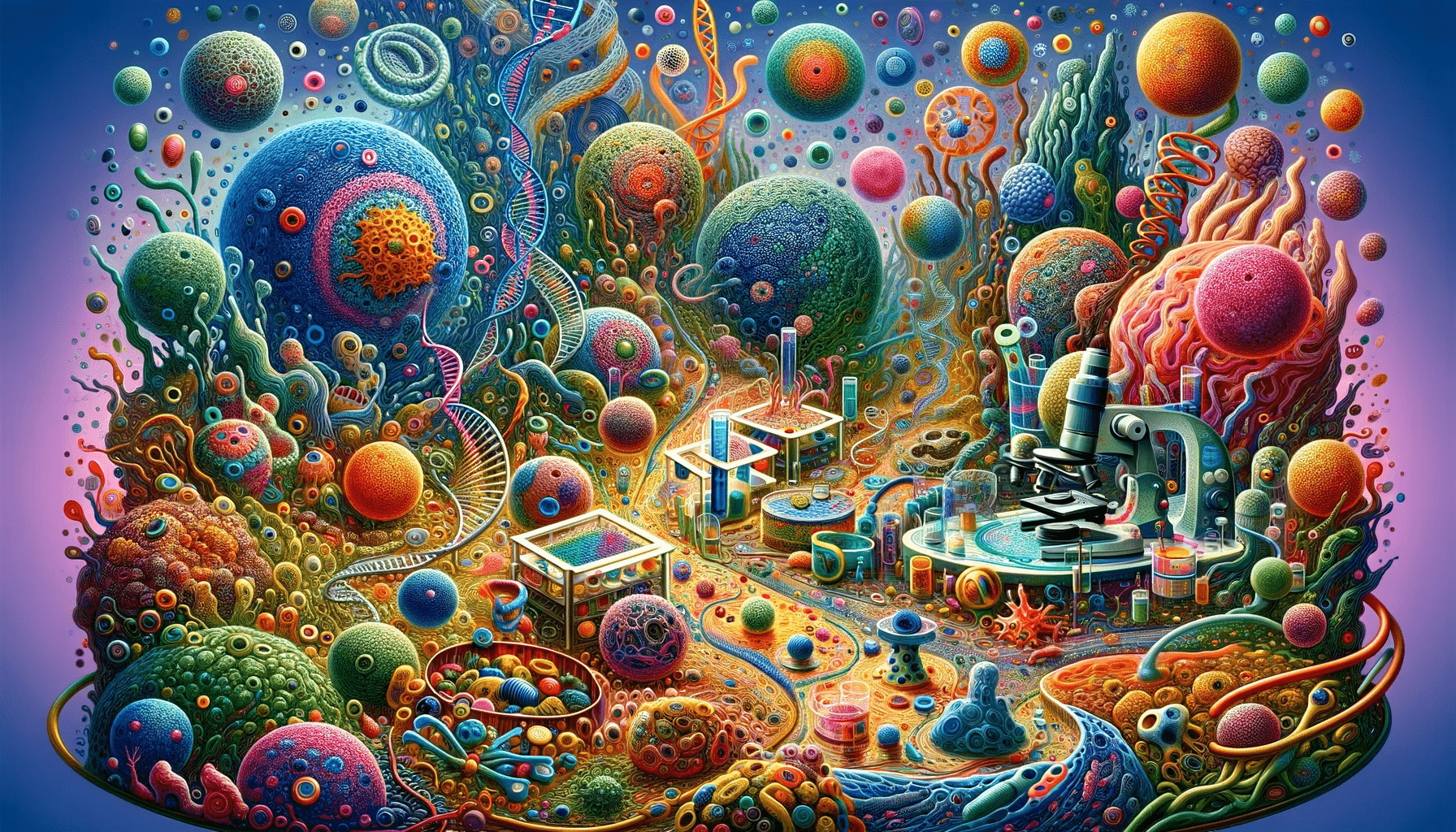This vibrant, digital painting, possibly AI-generated or computer-illustrated, depicts a fantastical, slightly sci-fi scene brimming with psychedelic colors. At its center is a floating planet-like structure surrounded by numerous cubes and spheres in vivid blues, oranges, pinks, greens, and yellows. Some of the cubes on the planet's surface contain test tubes, suggesting a scientific theme. Among the intricate, organic-looking roads and buildings, there is a prominent microscope that initially appears as a fountain. Additional vats of colorful liquid and rope-like objects are interwoven throughout the scenery, giving it the appearance of a futuristic laboratory city. The background features a gradient of blue and purple or blue and pink, enhancing the surreal, detailed artwork. The presence of planetary spheres and double helixes adds to the image's intricate, abstract aesthetic.